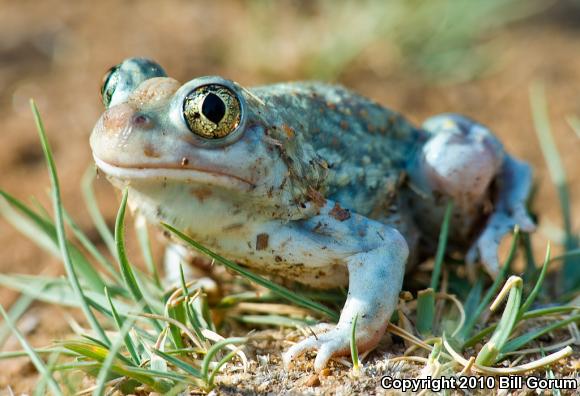The image captures a close-up of a frog situated in an outdoor setting with a blurred background. The foreground shows a patch of long grasses and brown dirt with some black rocks scattered about. The frog is uniquely detailed with an aqua blue back accented by hints of green and brown. Its legs and underside are predominantly white, with some debris and wood chips clinging to its body. The frog's eyes are distinctive, featuring golden rims, black centers, and a greenish hue encircling them. It appears to be facing slightly to the left, showcasing its prominent nostrils and curved mouth that gives it a contented expression. The image is watermarked on the bottom right corner with the text "Copyright 2010, Bill Goran."